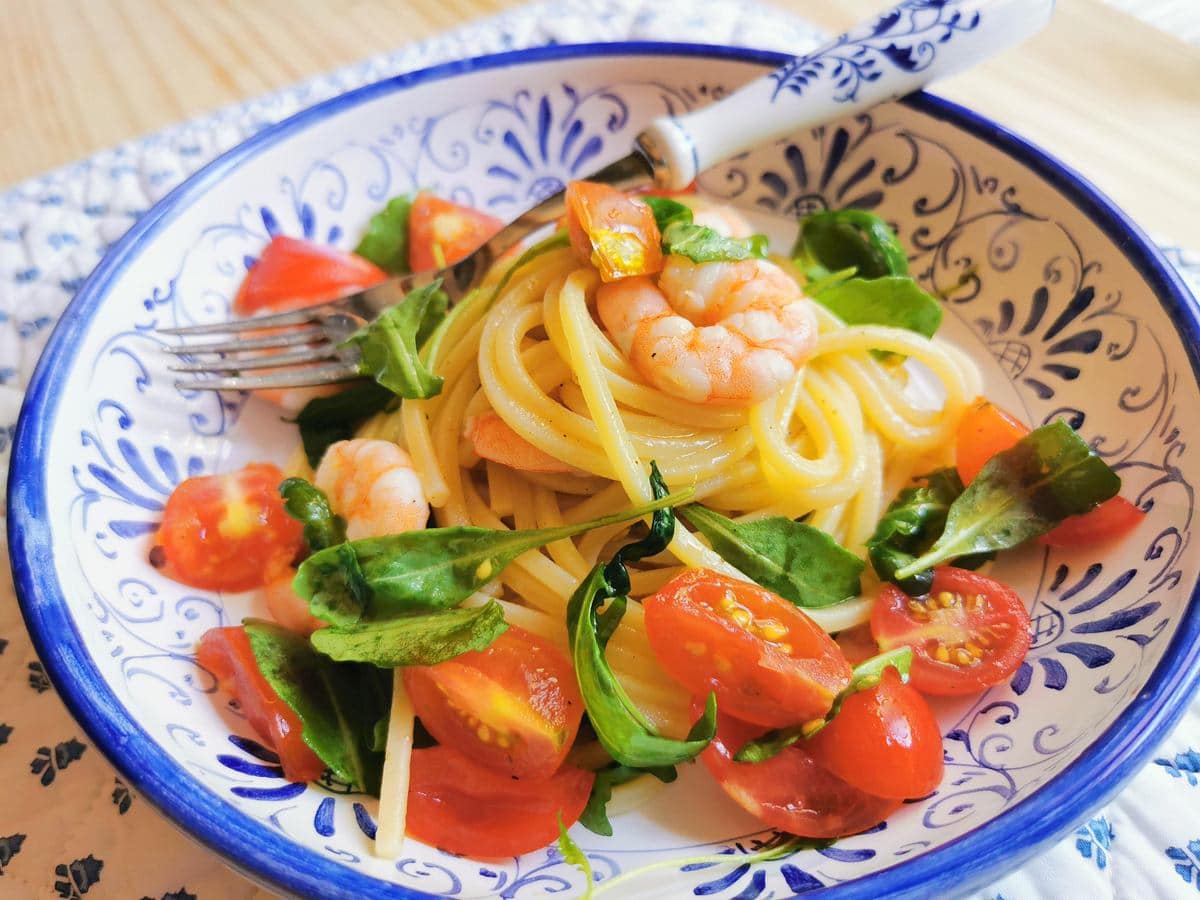In the image, there's a close-up of a beautifully plated pasta dish. This dish is served in a bowl with a blue rim and a white interior, featuring an ornate blue filigree pattern around its edges. Piled at the center of the bowl is a mound of yellow spaghetti, dressed in a light oil that gives the vegetables a glossy sheen. Atop the spaghetti, there are light pink shrimp, some of which curl over the pasta, while a mix of bright red cherry tomato slices and fresh green basil leaves are scattered around. A metal fork with a white handle rests on the far side of the bowl, adorned with a matching navy blue floral pattern. This entire setup sits on a white and blue placemat, placed on a light wooden table, visible in the top corners of the image.